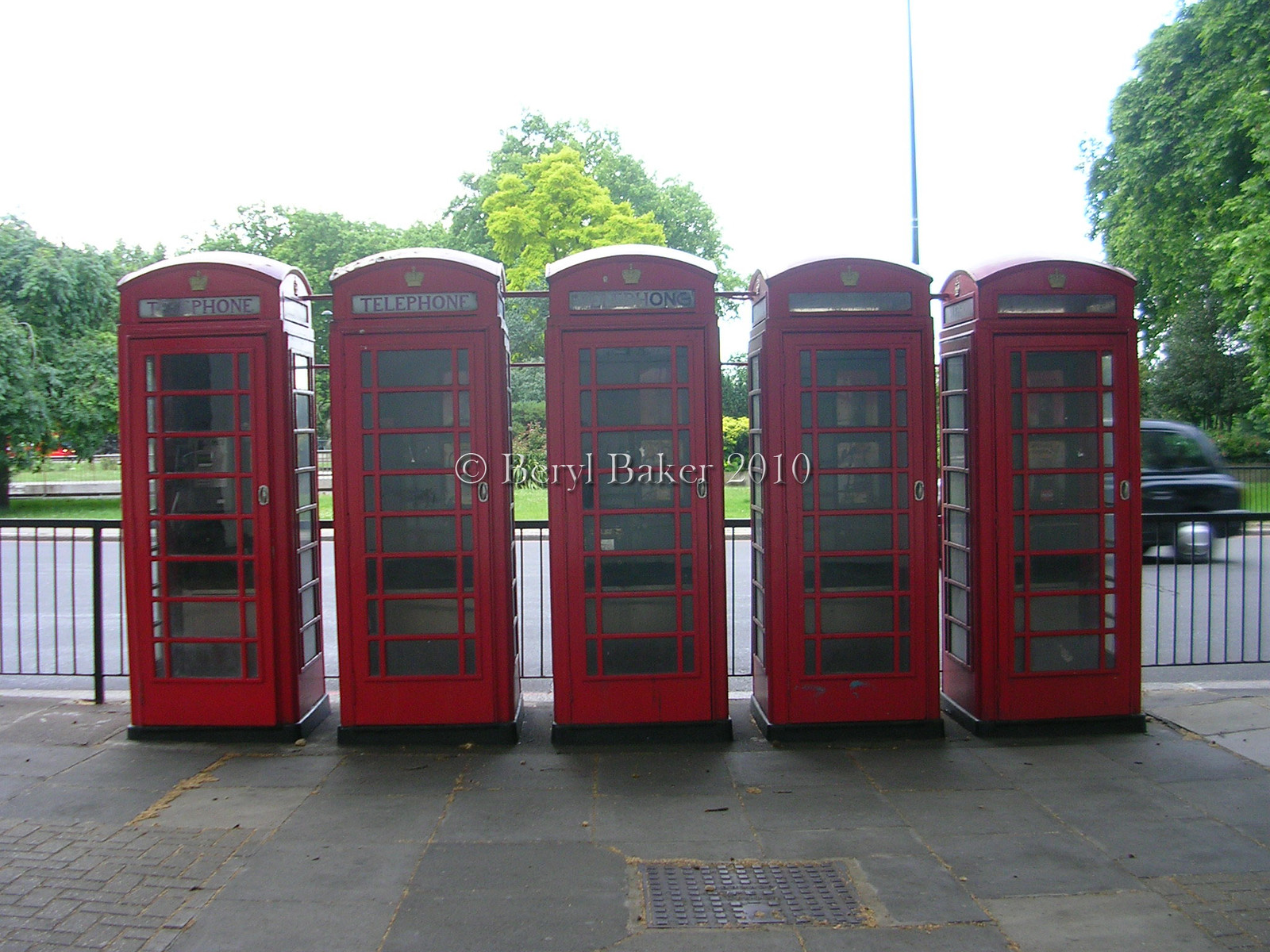This vibrant color photograph captures a quintet of British red telephone boxes standing in a line on a dark grey pavement just in front of a road. The iconic red booths are shadowed, each featuring golden crown emblems at the top and the word "TELEPHONE" in black on white panels - although some of the signs are partially missing or entirely absent. The structures boast classic glass doors partitioned by red bars. The pavement beneath them is dark grey, and there's a grate drain visible in the road before them. To the left corner, a smaller paved area is noticeable. A black metal fence with railings separates the sidewalk from the road. Behind the first telephone box on the right, the back of a black car, resembling a vintage London taxi, is visible. The scene is framed by a lush backdrop – a green tree line along with some yellowing leaves, with the sky a light whitish hue above it all. Intersecting the fourth telephone box, a slender spire extends upward into the sky, adding a touch of architectural intrigue.